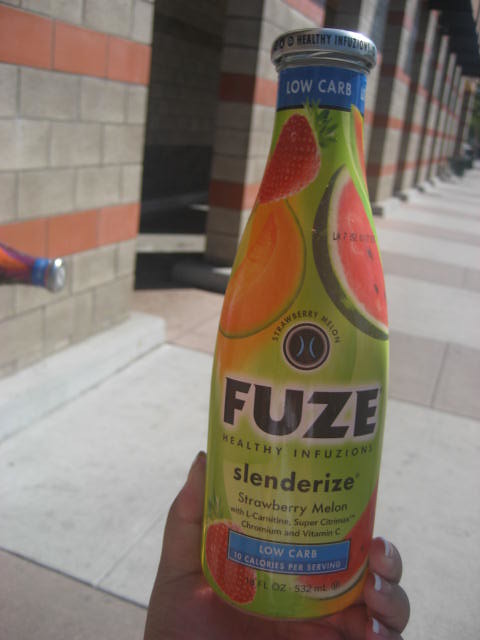In this vibrant image, a hand is prominently holding up a sleek, glass beverage bottle with a distinctively long neck and a small silver cap. The bottle itself is predominantly lime green and features colorful illustrations of various fruits - including a slice of watermelon, a whole strawberry, and a segment of mango - adorning its design. At the center of the bottle, the labels read "FOOS," "Healthy Infusions," "Strawberry Lemon," and "Low Carb" in a clean, modern font. The setting of the image includes a background featuring a light gray brick building with striking red stripes running horizontally across it. Below, the concrete sidewalk is visible, matching the light gray tones of the building and adding to the urban aesthetic of the scene. Overall, the image juxtaposes the vibrant, healthy drink against a muted cityscape backdrop, making the bottle’s lively design stand out even more.